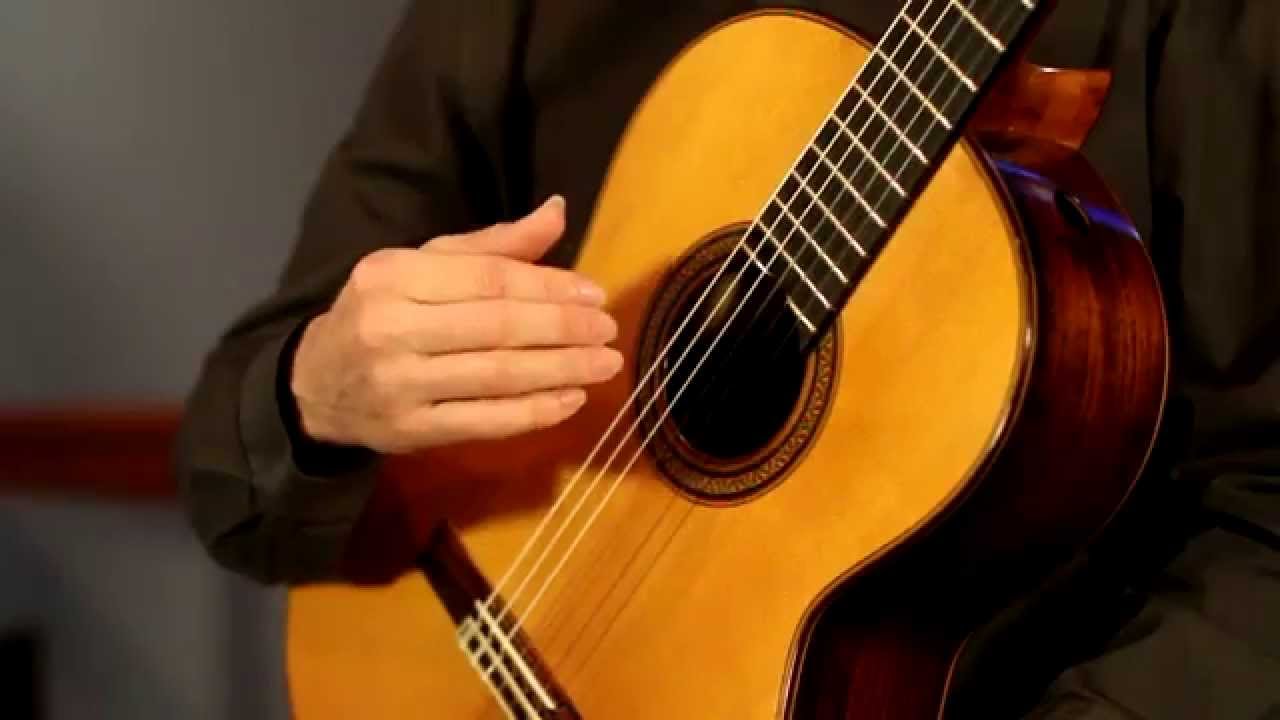This highly detailed photograph captures a close-up view of a person playing a six-string guitar. The focus is on the right hand, which is poised just above the strings, possibly preparing to strum. The hand, featuring longer fingernails, suggests the person might be a woman, although one account identifies the subject as a man. The individual wears a long-sleeved, dark olive drab shirt, not adorned with any jewelry. The guitar itself showcases a beautiful contrast with a blonde wood face and darker-stained wood on the sides, possibly cherry wood, oak, or hickory. The sound hole features a darker wood circle. The guitar lacks a pick guard, indicating it is designed to be played without picks. The background is softly blurred, presenting a gray wall with a wooden chair rail. Only a small segment of the surroundings is visible, enhancing the guitar and hand's prominence in the composition.